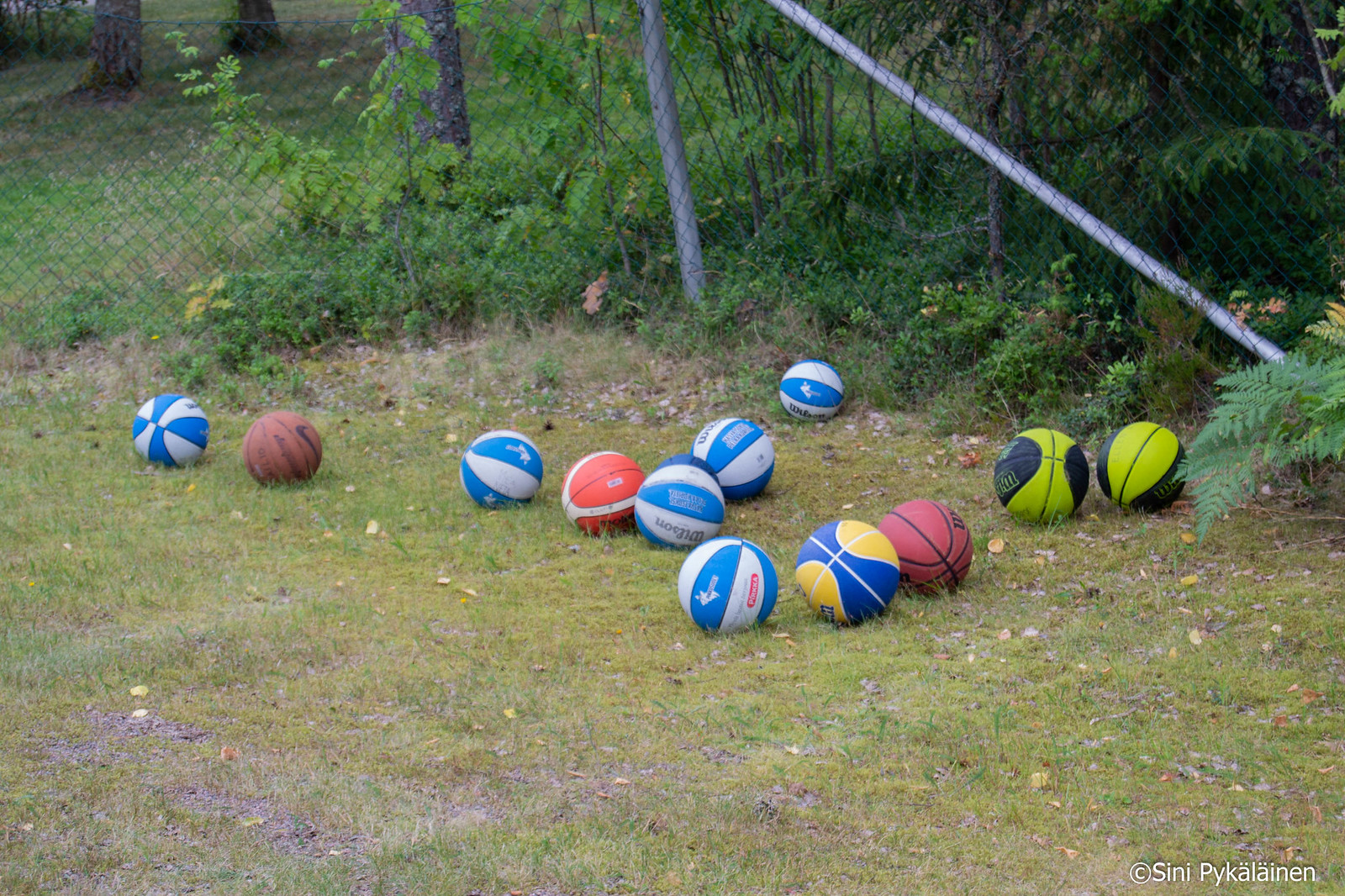This image depicts a well-maintained grassy soccer field with a soccer net prominently featured. The grass is short and light green, and in the background, there are trees and plants growing wildly. The soccer net, set against a backdrop of lightly overgrown greenery and a chain-link fence, has a triangular pole descending on the left-hand side and stretches with netting off to the right.

Scattered on the grass near the net, there are numerous balls, totaling around 15 in various colors and designs. Among these, there are ten soccer balls, five of which are baby blue and white with red lettering reading "Wilson." These five blue and white soccer balls are mostly grouped in the center, forming a pattern where four are aligned in a row to the left and one to the right. An orange ball with white stripes rests between these two clusters. 

Additionally, the image includes two traditional orange basketballs, an orange and white basketball, a blue and yellow ball, and two larger black and yellow balls also branded with "Wilson." There are also two green and black patterned balls. Amidst this array of balls, one stands out with a Nike swoosh logo. 

The scene appears reminiscent of a backyard playground, with the variety of sports balls scattered as though left there casually. There is also a noticeable piece of text at the bottom in white font that reads "Cini PYKA LAIN."